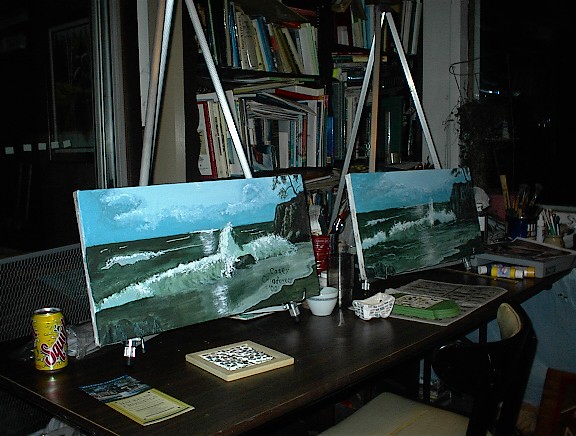This photograph captures the essence of an artist's studio, meticulously detailed and rich in character. Centered on a dark-stained wooden desk are two nearly identical beach-themed paintings, each poised on separate short desk easels. The paintings vividly depict waves crashing onto the shore with intricate differences; one features a misty wave with a notable gap in the front, while the other has a more defined, rock-crashing wave against a sunny backdrop. To the left of one painting sits a can of Squirt, adding a casual touch to the scene.

On the right side of the desk, organized containers hold an array of paintbrushes and other art supplies. The desk itself also has a few books and pamphlets scattered upon it, hinting at the artist's inspirations or references. Behind the desk, prominent and overflowing bookshelves house a diverse collection of books, suggesting a well-read and resourceful artist. An old-fashioned wooden chair with padded back and seat cushions stands ready at the desk, providing a comfortable spot for the artist to work.

Adding a final touch of ambiance, a window in the background allows natural light to fill the room, merging with the creativity and tranquility of the studio. This detailed scene perfectly encapsulates the artist's haven, a space where art and life beautifully intertwine.